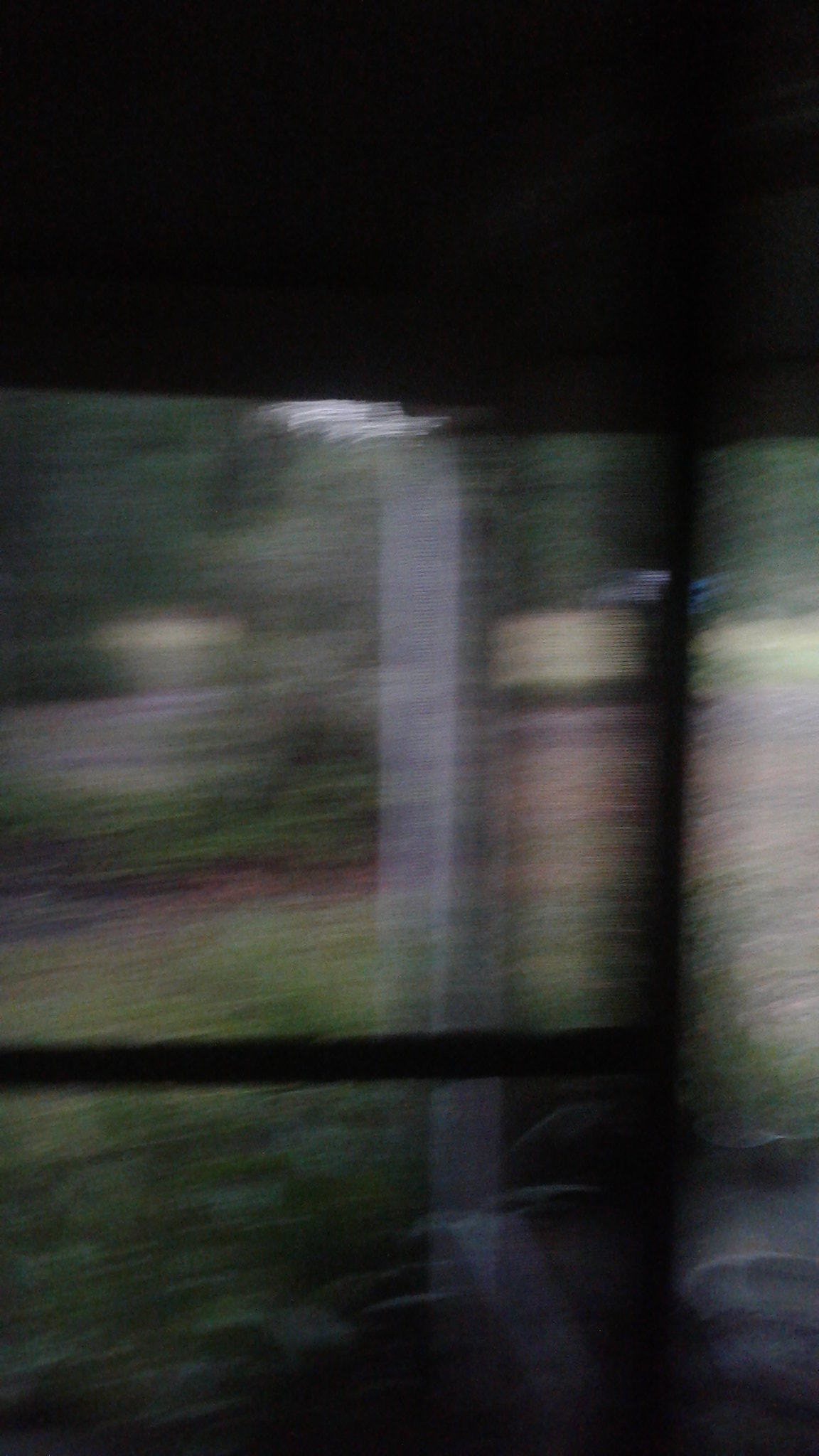The image is a blurry, low-light photograph taken from inside looking outside, likely through a window, giving it an out-of-focus and distorted appearance. The top 20% of the image is solid black, suggesting it was taken in the evening or in a dark location. A horizontal black line runs across the image, indicative of a window frame or screen. The scene outside is a mix of muted pastel shades, including greens, beiges, pinks, and grays. The right-hand side features what look like two cylinders, which are colored in bands from green at the top, yellow, pink, green again, and ending in gray. The background out the window displays greenery, possibly grass and bushes, and objects that could be a concrete pole and a bowl or pot. The overall impression is of a slightly surreal, motion-blurred view with a jet-black upper section, streaks of white, and a mix of pastel colors all blending together in the lower sections.